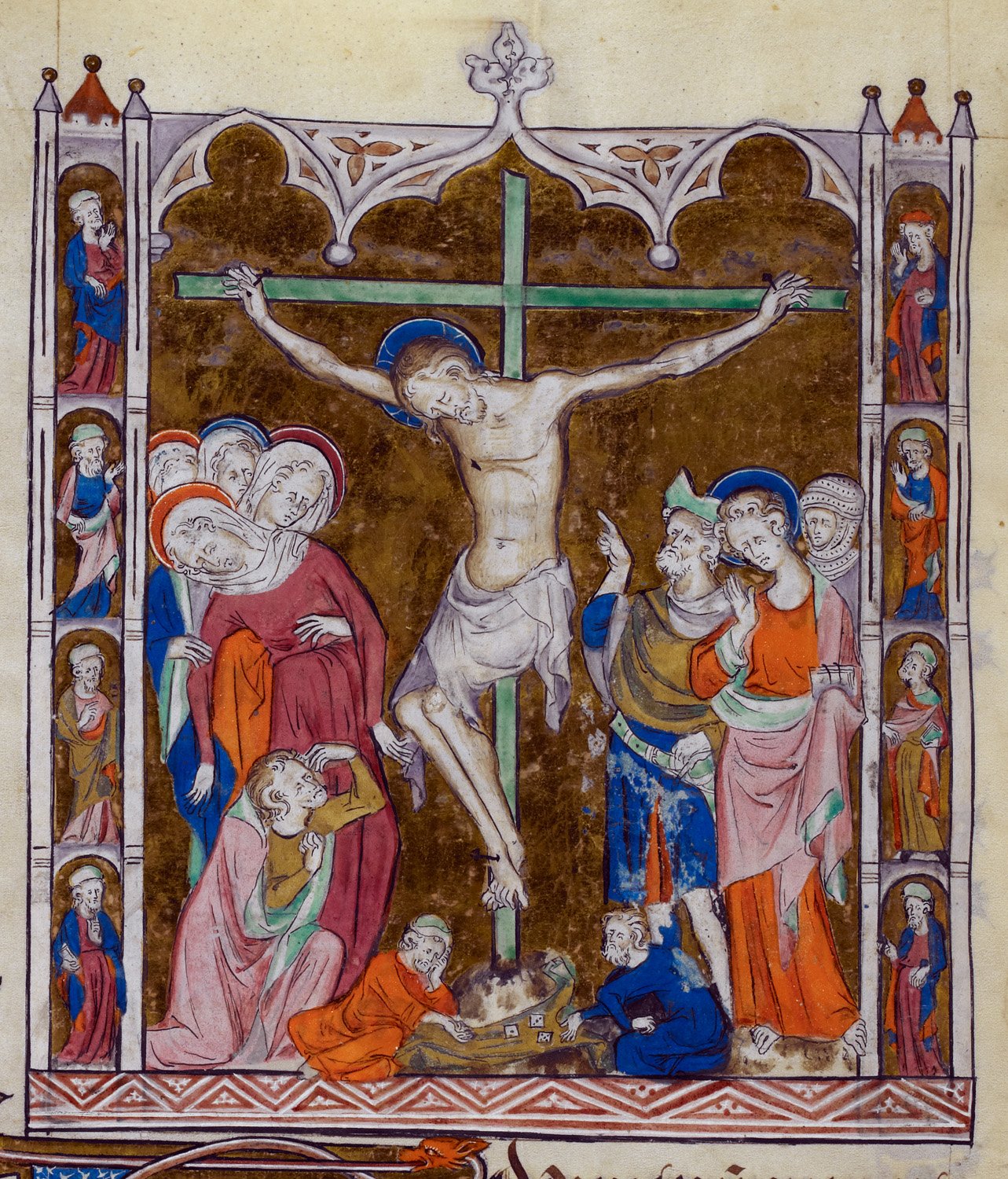This rectangular image, taller than it is wide, appears to be an intricate vintage painting or colored drawing depicting the crucifixion of Jesus. Central to the composition is Jesus on a thin, green cross, his head tilted to the left, with a white fabric draped around his waist. Surrounding him on both sides are disciples adorned in flowing robes and head coverings in shades of orange, blue, and red. Below him, at the foot of the cross, sits a baby and the upper part of a reddish-brown dog’s head. To the right, a bearded man raises his right arm, pointing upward towards Jesus.

The background of the scene is primarily brown, with a black area providing contrast. The image features ornate borders with arches and columns resembling a castle structure, framing the central crucifixion scene. There are multiple smaller scenes within the main image, each depicting various disciples in different postures, some sitting and some standing, enhancing the narrative depth. At the bottom of the illustration is a geometric design of cream and reddish triangles, adding to the decorative detail. The entire artwork is set against a backdrop of gray and cream, evoking the feel of an ancient, cherished manuscript.